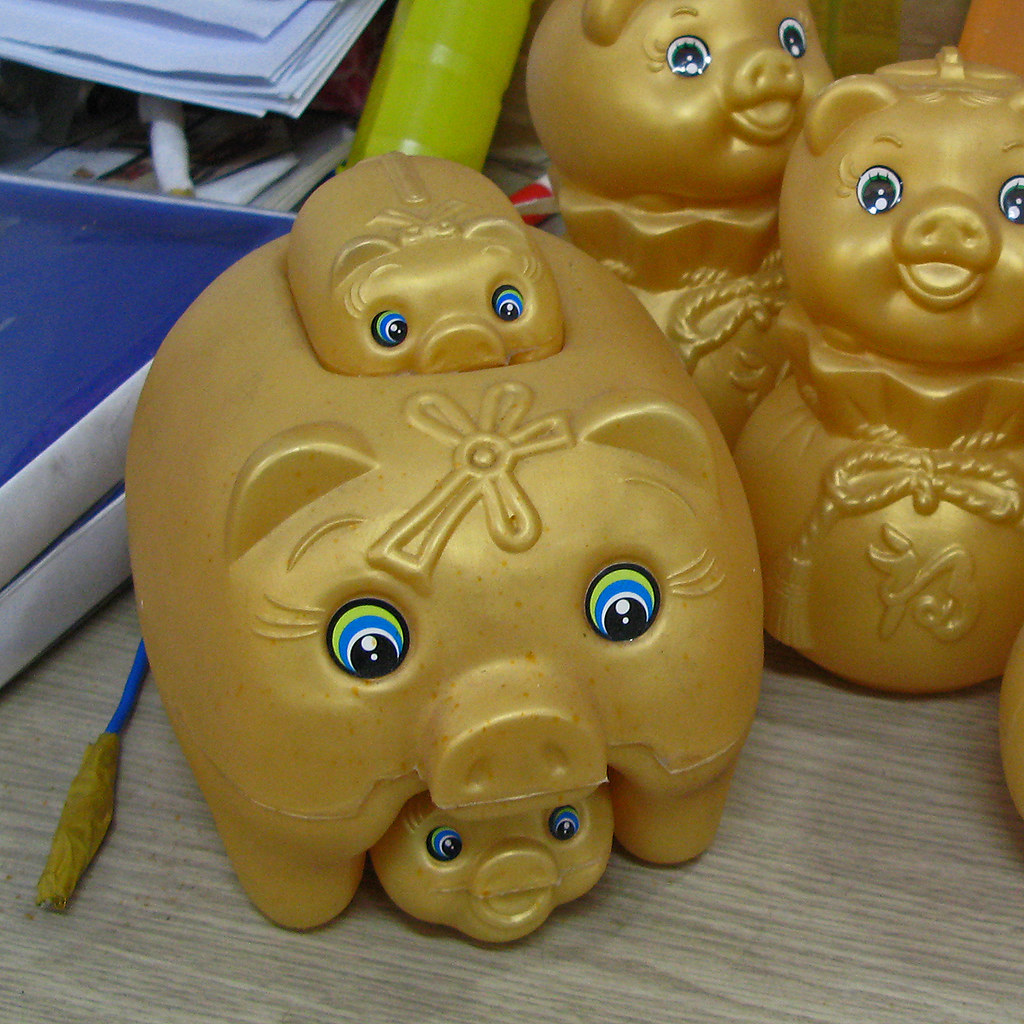In this photo, set on a wooden table with a vertical grain, we see a collection of golden pig figurines, detailed with blue and green eyes featuring white dots in the center of their black pupils. The focal point is a large piggy bank with a ribbon on its head, whose molded plastic features include eyelashes, eyebrows, a snout, and the distinctive multicolored eyes. Attached to the bottom of this main pig is a baby pig, while another baby pig appears squished into an indent on its back.

To the right, there are additional golden piggy banks resembling pig heads poking out of a sack, complete with a molded rope and a Chinese character on the surface. These pigs also have eyes, primarily black with less pronounced green and blue. Additionally, behind these piggy banks, we can spot a blue tray with a white border, a stack of white papers, and what appears to be a green plastic tube or possibly a paintbrush with a blue handle.